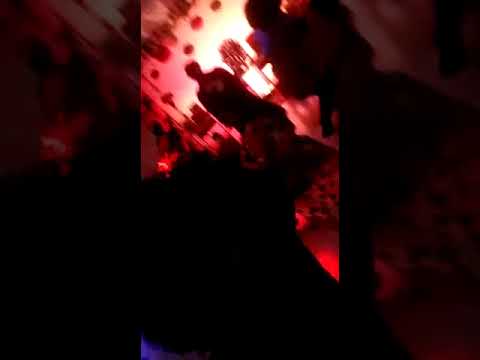The image is a realistic photograph set inside a darkly lit bar or nightclub. It is the center panel of a triptych, with black panels on the left and right sides. The photo is oriented at a 90-degree tilt, causing the people to appear diagonal. The most visible person is a woman wearing a black and white dress, standing prominently in the foreground. Next to her is an individual with frizzy, afro-style hair, dressed in a blue shirt and dark or black pants. Behind this person, there's a woman seated in the background. The farthest background features a wall adorned with red polka dots or similar decorations, illuminated by a yellowish-reddish light, which contributes to the dim lighting of the room. Another indistinct shape, likely a person, is visible behind the woman in the dress. The image captures a lively social setting, despite the challenging lighting conditions. There is no text present in the image.